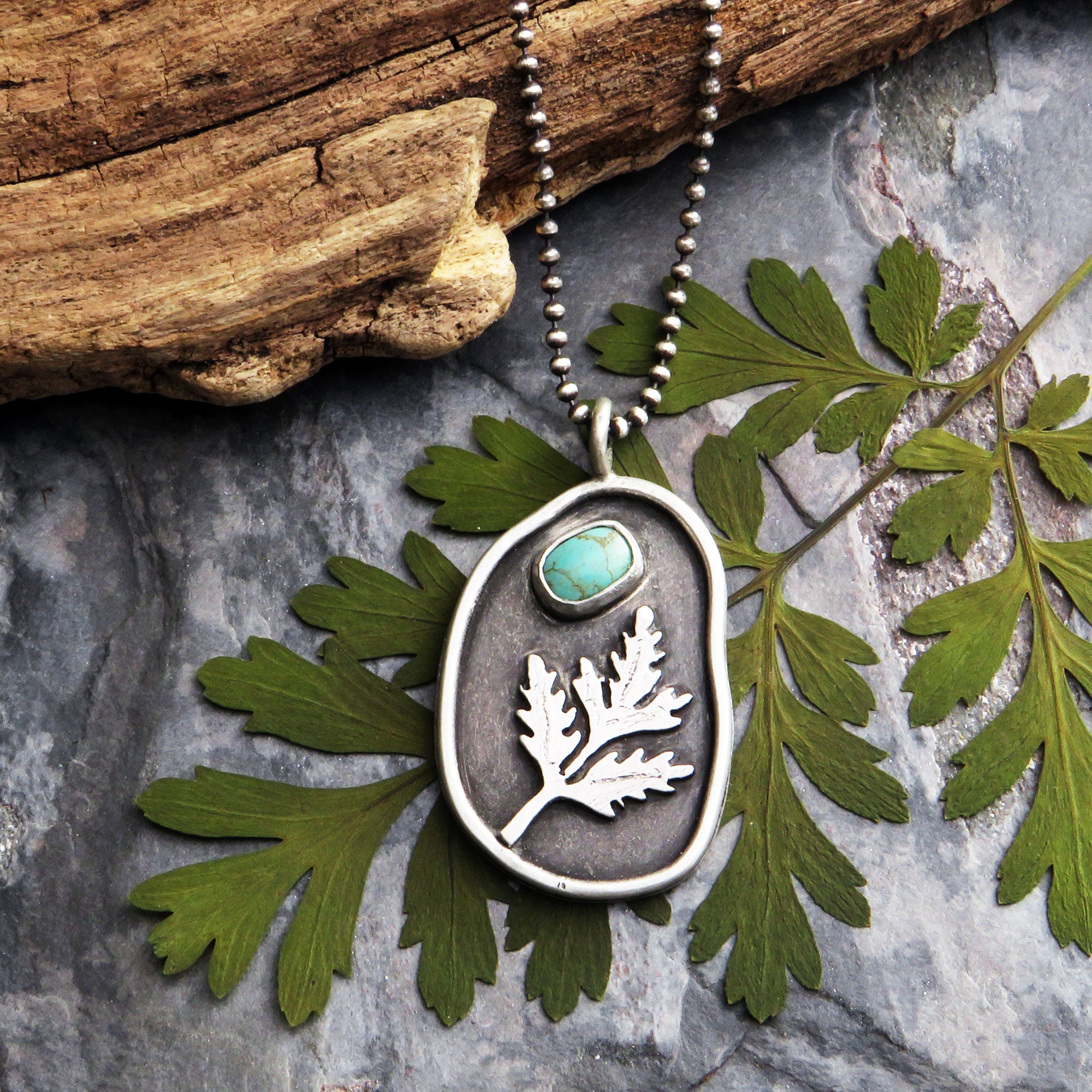This photograph showcases a beautifully crafted silver necklace, likely available on a platform like Etsy. The background features a textured dark grey marble, lending an earthy and natural ambiance to the image. At the top of the picture, a piece of driftwood is draped with a delicate silver ball-and-chain. The focal point of the image is the silver, egg-shaped pendant that contains a raised silver leaf. Positioned above the leaf is a striking turquoise stone with veins of brownish-gold, adding a vibrant pop of color. Underneath the pendant lies a flat, previously live leaf, which mirrors the fern depicted within the necklace. This arrangement enhances the organic, nature-inspired theme of the jewelry piece. The necklace and its intricate setting suggest a handcrafted design, perfect for artisan jewelry enthusiasts.